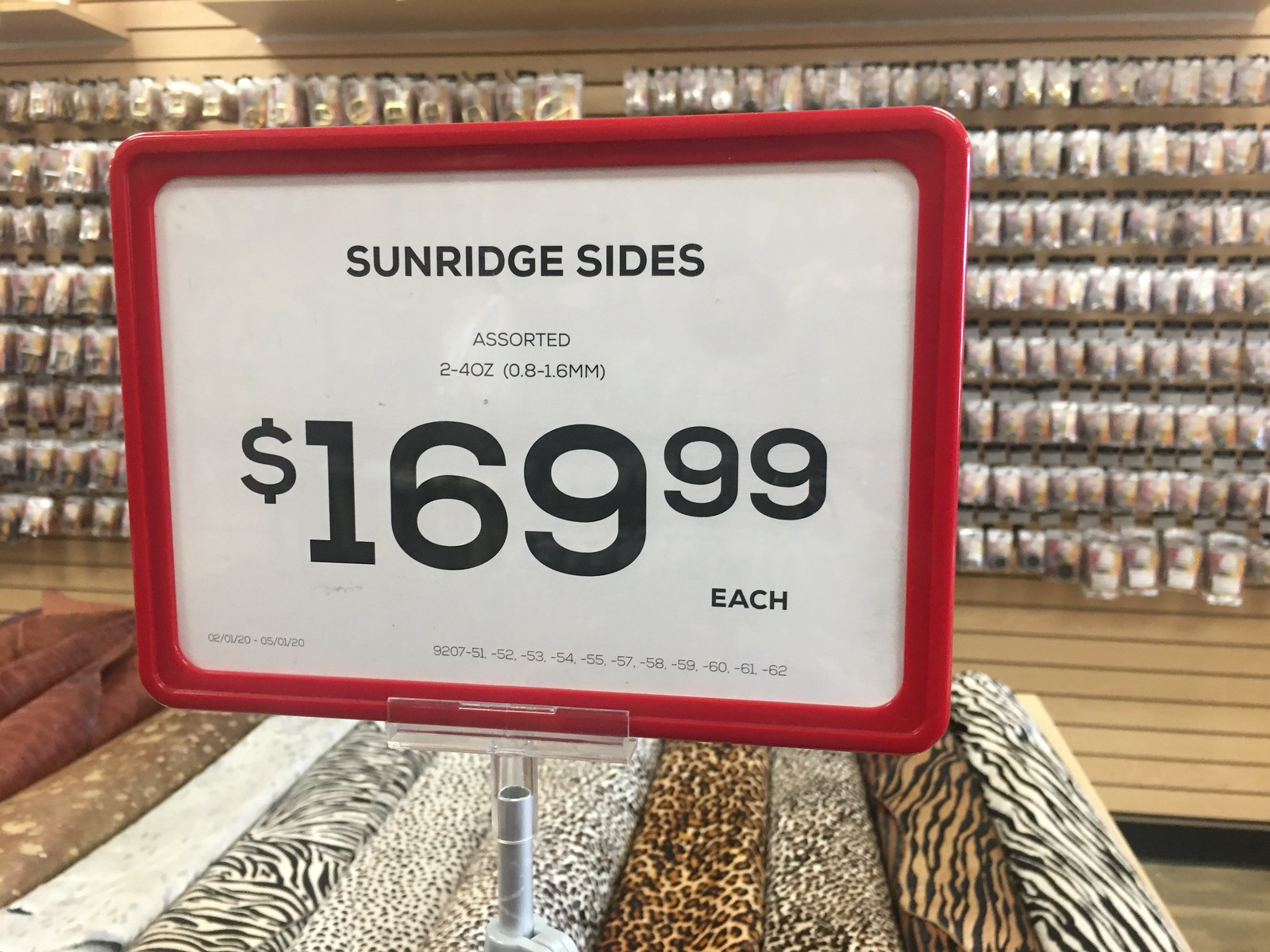Inside the store, a rectangular sign with a large red plastic frame takes center stage in this horizontal image. Positioned on a mount or small stand, the sign rests atop several rolls of fabric, each showcasing various animal prints in shades of black and white. The vibrant patterns include tiger stripes, cheetah spots, and zebra lines, along with some plain designs. The sign reads: "Sunridge Sides - Assorted 2-4 oz. (0.8-1.6 mm) $169.99 each," and includes the date range "01-20 to 05-12-20." In the background, a horizontal-paneled wall is adorned with rows of metal hooks, holding an array of packaged items across eight distinct rows. The detailed patterns and organized display create an engaging and visually appealing scene inside the store.